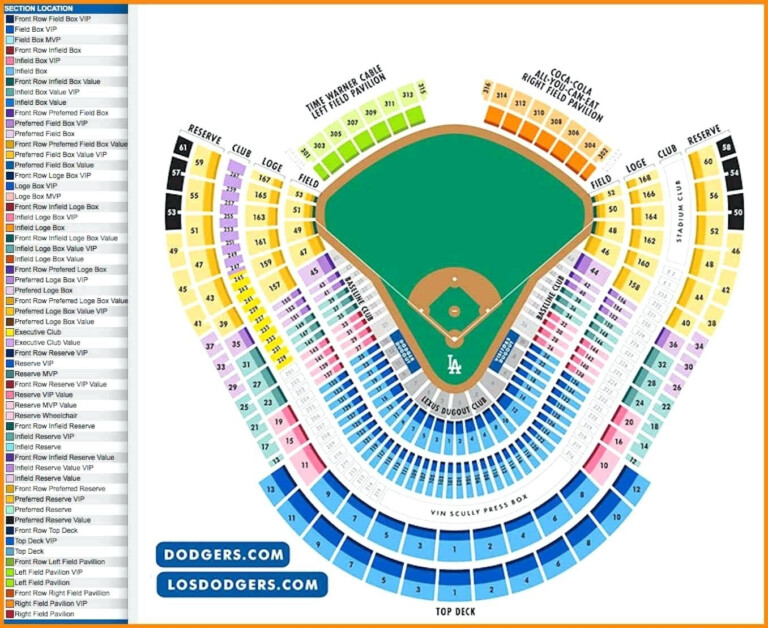This detailed seating map of Dodger Stadium is meticulously outlined in orange against a pristine white background. Dominating the left side of the image is a comprehensive menu headlined "Section Location." This menu features at least 20 small, color-coded boxes, each labeled with the corresponding seating areas. The central focus of the map is an overhead view of the baseball field, resplendent in vibrant green and framed by a brown dirt outline. Directly behind home plate, the iconic LA logo of the Los Angeles Dodgers is prominently displayed. The seating arrangement forms a U-shape around the front of the diamond, with different sections marked in various colors that correspond to the menu on the left. In the bottom left corner of the image, two blue buttons, inscribed with white text, read "Dodgers.com" and "LostDodgers.com," providing convenient links for more information.